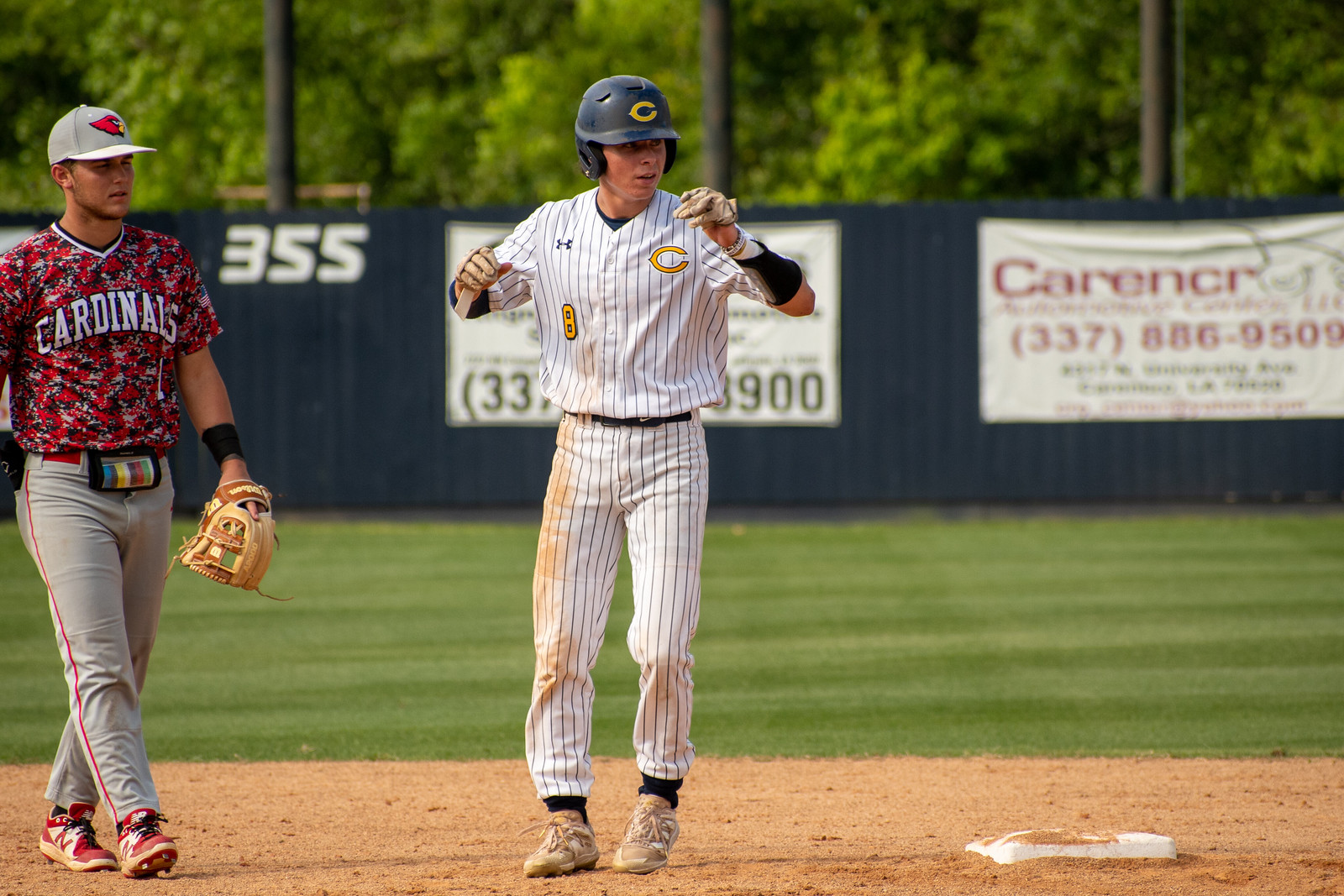In this outdoor photograph taken on a pleasant day, two baseball players are standing on the dirt part of a baseball diamond with a base visible in the bottom right corner. The player to the left of the base is wearing a Cardinals uniform, including a red and black camo-patterned shirt that says "Cardinals" in white font, gray pants with red accents, red shoes, and a cap with a Cardinal logo. He also has a baseball mitt in his left hand and is facing slightly to the right. To his left stands another player, dressed in a Cubs uniform, which consists of a white jersey with thin black lines, a black helmet, and a black cap, both featuring a yellow "C." This player is looking to the right. The background of the image includes a tall, dark blue fence adorned with signs and advertisements. One sign on the right reads "Carencer" along with a phone number, while another sign near the center, partially obscured, shows the number "355." The top of the image reveals some trees and leaves, adding a natural touch to the scene.